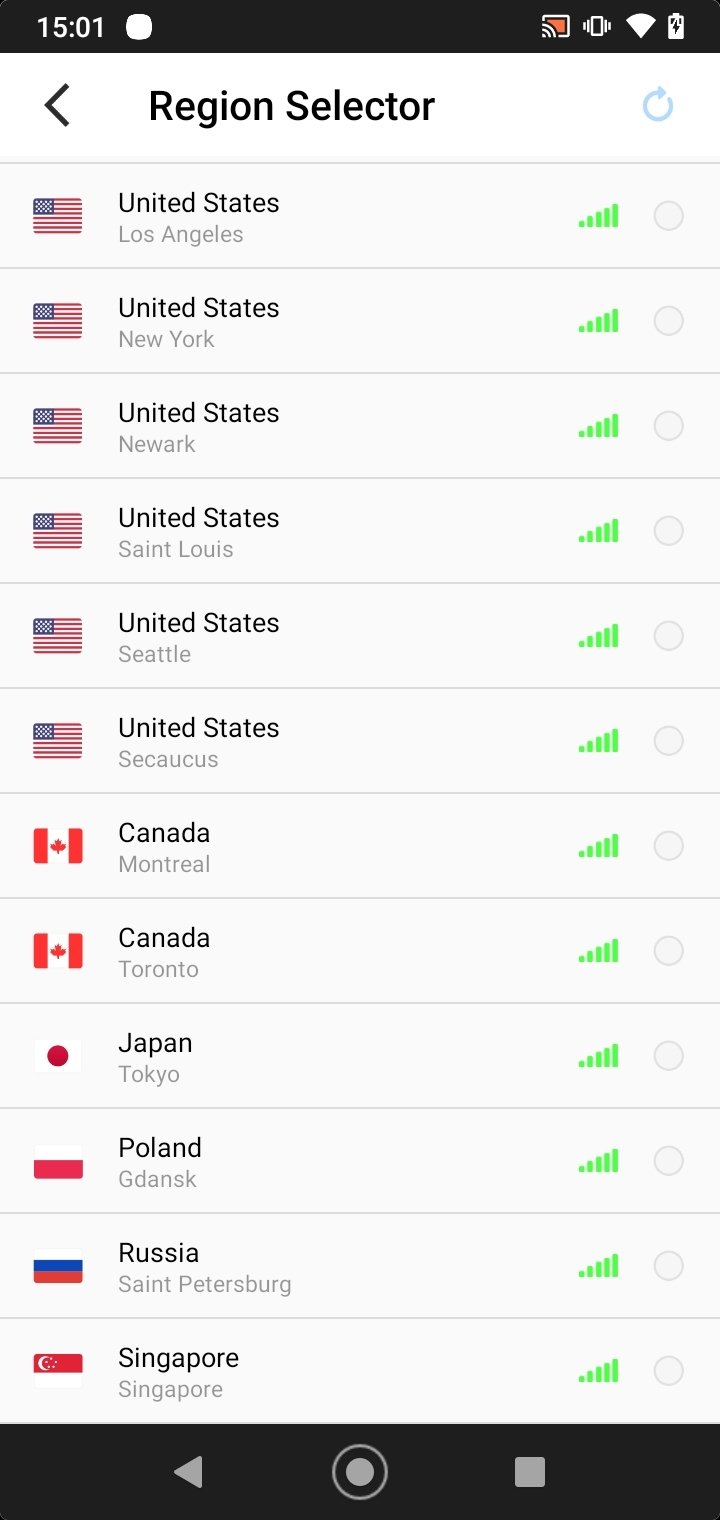This image is a mobile screenshot of a region selector page. The interface has a clean design with a white background. At the top left, there is a prominently large, black arrow pointing left, indicating a way to go back to the previous screen. Centered at the top is the text "Region Selector" in bold black font, flanked on the far right by a light blue refresh icon.

The body of the page features a vertical list of regions on the left side, each accompanied by their respective signal strength indicators and selection bubbles on the right. Each region entry is formatted in the following way:

1. At the top, the first entry shows the United States with a flag icon to the left. "United States" is written in bold black letters, and below it, "Los Angeles" is displayed in gray font. Adjacent to this, on the right side, small icons represent a full five-bar signal strength and an unchecked click circle.

2. The second entry mirrors the format with the United States flag icon followed by "United States" in bold black letters, and below it, "New York" in gray. This entry also shows a full five-bar signal strength and an unchecked click circle.

Further entries continue in a similar pattern, listing various regions with their respective icons, subordinate cities, signal strength indicators, and clickable selection circles. The final entry at the bottom of the list is for Singapore, with its respective flag icon, region name, and full signal strength. Like the others, Singapore is not selected.